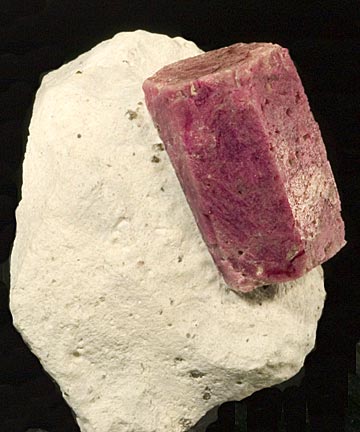In a photograph set against a solid black background, two distinct rocks seemingly float in a black void. The larger rock, which occupies the rear part of the image, is creamy white with a few gray spots and numerous small pits across its mostly smooth surface. This rock is rounded, without any jagged edges, and exudes a natural, eroded appearance often attributed to calcium deposits. In contrast, the smaller rock in the foreground is roughly half the size of the larger rock and is characterized by its hexagonal, cylindrical shape. This smaller rock displays a unique pinky-purple hue, with some describing it as rosy maroon or a blend of red and brown. Both rocks appear intricately meshed together, creating a striking compositional balance within the stark, empty backdrop.